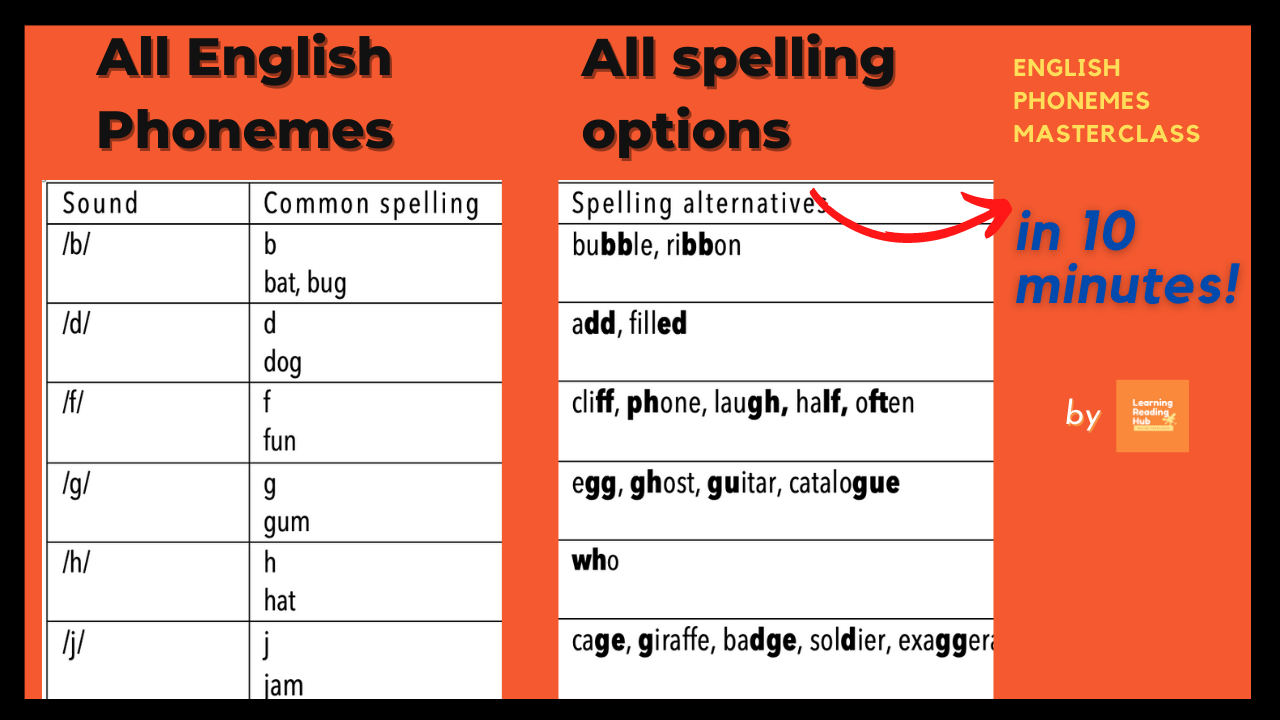The image depicts a classroom advertisement laid out in chart form, bordered in black with a prominent orange background. The left side of the chart outlines various English phonemes, with corresponding sounds and common spellings listed in white text. Examples include sounds for B (/b/) with spellings such as "bat" and "bug," D (/d/) as in "dog," F (/f/) as in "fun," G (/g/) as in "gum," H (/h/) as in "hat," and J (/j/) as in "jam." Adjacent to this chart, a detailed list of alternative spellings is provided, featuring words like "bubble," "ribbon," "filled," "cliff," "phone," "giraffe," and "exaggerated." The top right corner of the advertisement highlights the phrase "English Phonemes Master Class" in bold yellow text, alongside a note in blue indicating that the content can be mastered in ten minutes. The overall design employs a vibrant mix of colors including orange, black, yellow, blue, white, and red to draw attention and aid in learning.